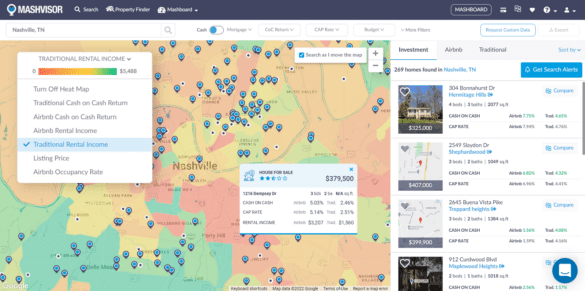Displayed is a screenshot of a rental property search interface, identified as MASH Visor. At the top, the header includes options such as "Search," "Property Finder," and another partially visible option that might read "MASH Board." Below this, a search bar shows a query for "Nashville, Tennessee," with the search filtered to display properties available for cash purchase. 

The main section on the left features a map of Nashville, color-coded to indicate traditional rental income ranges from $0 to $5,488. The gradation spans from red (lower income) to blue-green (higher income). The map visually represents different regions of Nashville based on rental prices, and the traditional rental income option is selected.

On the right side, a panel lists 269 homes found in Nashville, providing details and markers for each property. This organized and user-friendly system enables users to effectively explore rental property options in Nashville, with clear visual cues and comprehensive property details to assist in the search process.